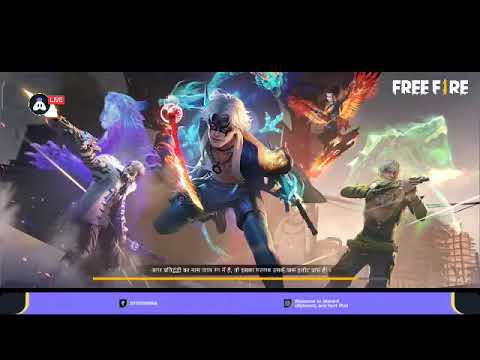In the image, which appears to be a screenshot or advertisement for the video game "Free Fire," dynamic and colorful elements highlight a scene featuring multiple characters and vivid backgrounds. The prominent text "Free Fire" is situated in the top right corner, with the "I" in "Fire" depicted as a gilded bullet. The visual is dominated by four distinctive characters each holding weapons and exuding a striking aura. The central character stands front and center, adorned with a black mask, white hair, a gold top, and blue pants, wielding two swords. To his left, a character aims a weapon, backed by a glowing purple spirit-like entity. On his right, another figure is accompanied by a tortoise-like spirit. Above this central figure, at approximately a 45-degree angle, a character with blazing red wings and a jet pack, resembling a phoenix, is seen mid-flight. The backdrop displays a derelict, gray-brown cityscape with blurred, destroyed buildings, casting a stark contrast to the vivid purples, reds, yellows, blues, and greens employed throughout the image. Below, a purple banner further intensifies the vibrant atmosphere. Overall, the image encapsulates the essence of an action-packed, superhero-themed 3D video game.